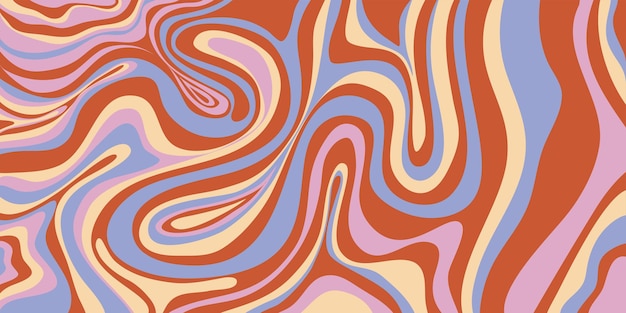The image is a computer-generated rectangular artwork characterized by an array of colorful swirls and patterns that evoke a groovy, retro vibe reminiscent of the 70s. The swirls, which intersect and touch each other in a seemingly random fashion, range in color from light blue and pink to brown, beige, and cream. The swirling motions suggest a chaotic yet artistic design, akin to paint being dragged and manipulated across a canvas with paintbrushes in various directions. The colors also include light purple, dark reddish hues, and orange, contributing to a lively, vibrant aesthetic that could easily adorn the wall of a trendy restaurant or mural. The swirling, squiggly lines and vivid color palette create a dynamic and eye-catching visual reminiscent of flower power era designs, making the artwork both visually engaging and nostalgic.